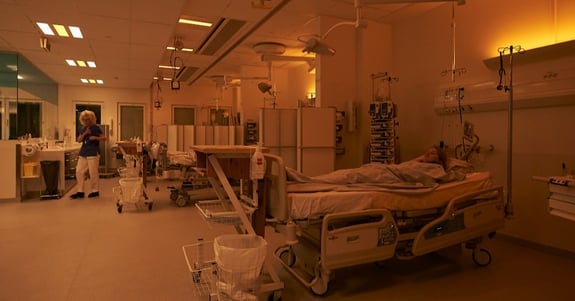The sepia-toned image depicts a dimly lit hospital room, with an overall orange hue dominating the scene. In the foreground, a woman is resting on a hospital bed, covered with a blue sheet against a white mattress. There's a tall stand and a trash can at the foot of her bed, likely where a doctor would update orders. An IV pole is also present, although it's not currently in use. On the wall above her, a light casts an orange glow. Further into the room, dividers section off different areas of the hospital, adding to the sense of partitioning. Near the background, a figure, possibly a nurse, characterized by blonde hair and dressed in a blue scrub top with white pants and black shoes, stands by a nurse's station. Various medical equipment and perhaps a couch or seating area are faintly visible in the dim lighting. The atmosphere suggests it could be a recovery center post-surgery.